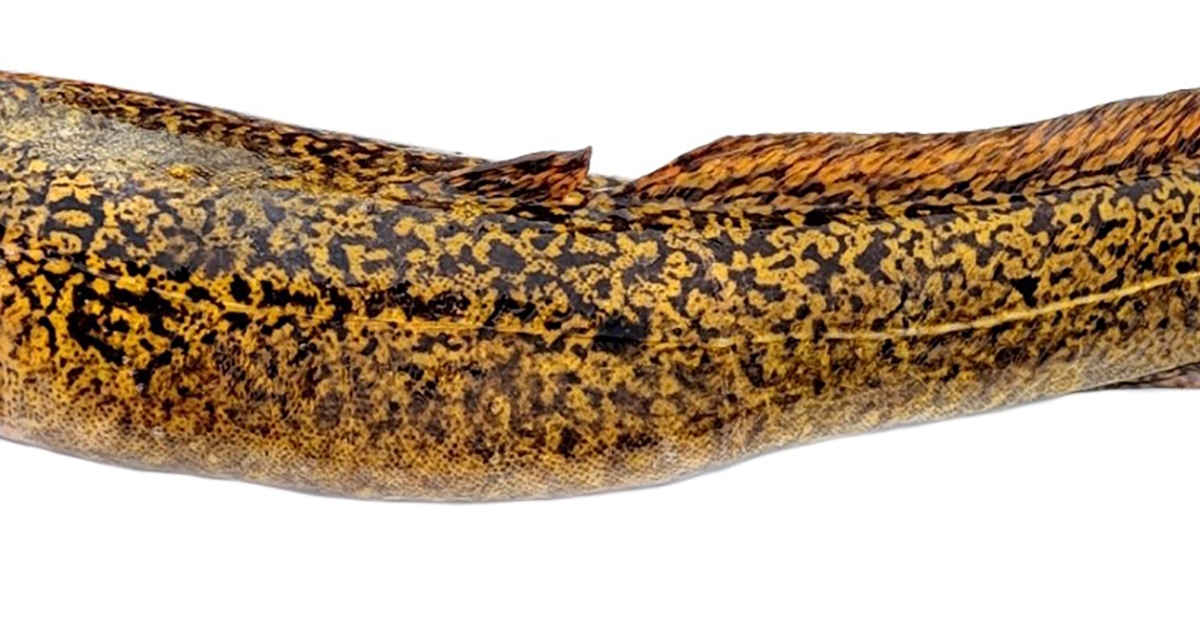The image showcases a close-up view of a textured, yellow and black patterned surface, likely representing the body of an eel or snake. The object extends across the entire width of the photograph, isolated on a perfectly white background, offering no contextual clues. Its skin appears textured with a distinct yellow and black pattern. Notably, there is an orangish ridge, about an inch high, running along the top of the body. Fins can be seen on the top right side, while the left side remains flat, suggesting the central portion of the animal's body is depicted. The image quality is average, and no text or additional features are present.